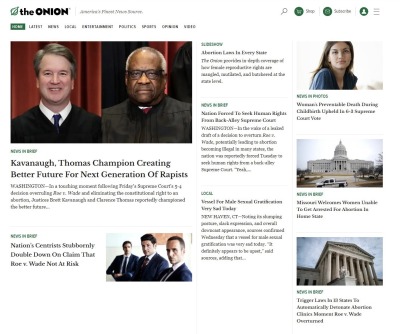The image features a page from *The Onion*. In the top-left corner, there's a small green leaf icon next to "The Onion," written in bold black text, followed by "Syndicated Press." Below this header, a green button is labeled, indicating sections like "Latest News," "Entertainment," and "Politics."

At the top of the page, a prominent image showcases Judges Kavanaugh and Thomas dressed in their traditional black judicial robes. The headline reads, "Champion Creating Better Future for Next Generation of Rapists," a satirical jab typical of *The Onion's* content.

Beneath this main image is another photograph depicting three men in black suits standing before a red and white flag. The accompanying text discusses the nation's controversial stance on Roe vs. Wade, suggesting that the ruling is now at risk.

Toward the middle of the page, three smaller boxes contain brief articles. On the right side of the page, there are three additional images. The first features a young girl, the second depicts what appears to be the Capitol Building under a clear blue sky, and the third also seems to be another angle or perspective of the Capitol Building. Each image is paired with respective articles, likely addressing various satirical takes on current events.